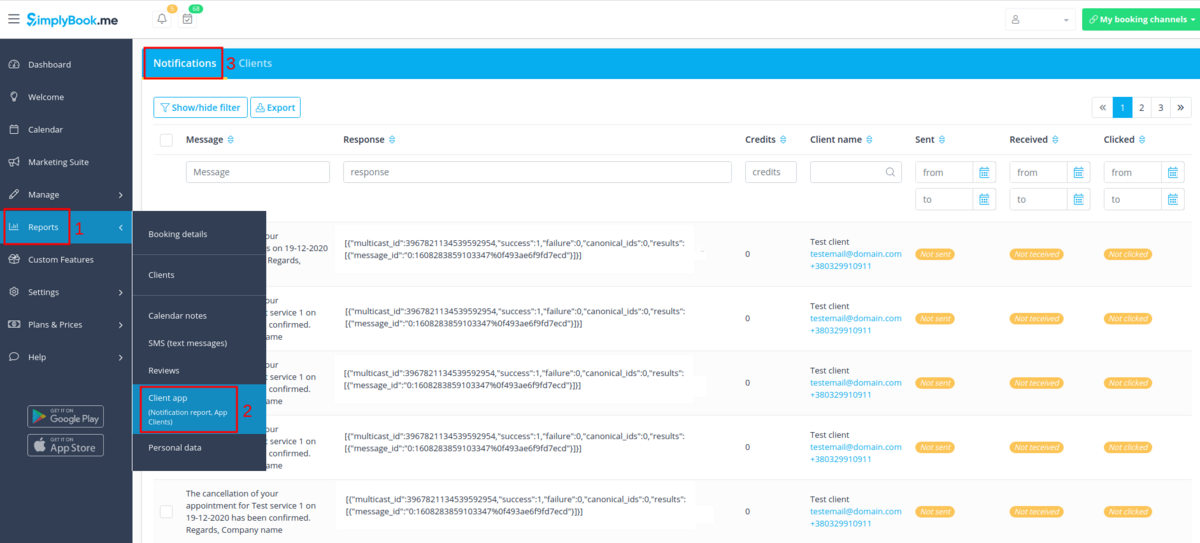The image showcases a computer screen displaying the interface of a bookings website called simplybook.me. In the top left corner, there are three horizontal bars representing a menu button next to the website's logo. Adjacent to these, a notification bell with a yellow alert icon and a calendar icon with a green event indicator are visible. 

On the right-hand side of the screen, a small person icon likely serves as a link to the user profile. Below it is a lime green rectangular button labeled "My Booking Channels" in white text.

Dominating the left side of the screen is a vertical navy blue sidebar featuring several menu options: Dashboard, Welcome, Calendar, Marketing Suite, Manage, Reports, Custom Features, Settings, Plans and Prices, Help, along with icons for downloading from the Google Play and App Store. The "Reports" section is selected, highlighted with a red rectangle around it and a red number one, indicating it is active.

A secondary pop-out menu shows sub-options such as Booking Details, Clients, Calendar Notes, SMS, and Reviews. The "Client Apps" option is currently selected, marked by a red rectangle and a red number two, with the "Personal Data" option listed below.

Just below the top bar of the screen is a large, light blue rectangular banner with white text labeled "Notifications and Clients." The "Notifications" option is active, highlighted with a red rectangle and a number three. There's also a "Show/Hide Filter" button and an "Export" button, both framed in light blue on a white background.

The main section of the screen displays a messaging interface resembling a spreadsheet, segmented into six categories: Message, Response, Credits, Client Name, Sent, Received, and Clicked. Five messages are visible, and the text is largely in small, difficult-to-read font. The entries appear to be from test clients, suggesting this may be a test environment.

In summary, the captured screen displays a detailed view of simplybook.me’s reporting section with various navigational elements and options for handling bookings and client communications.